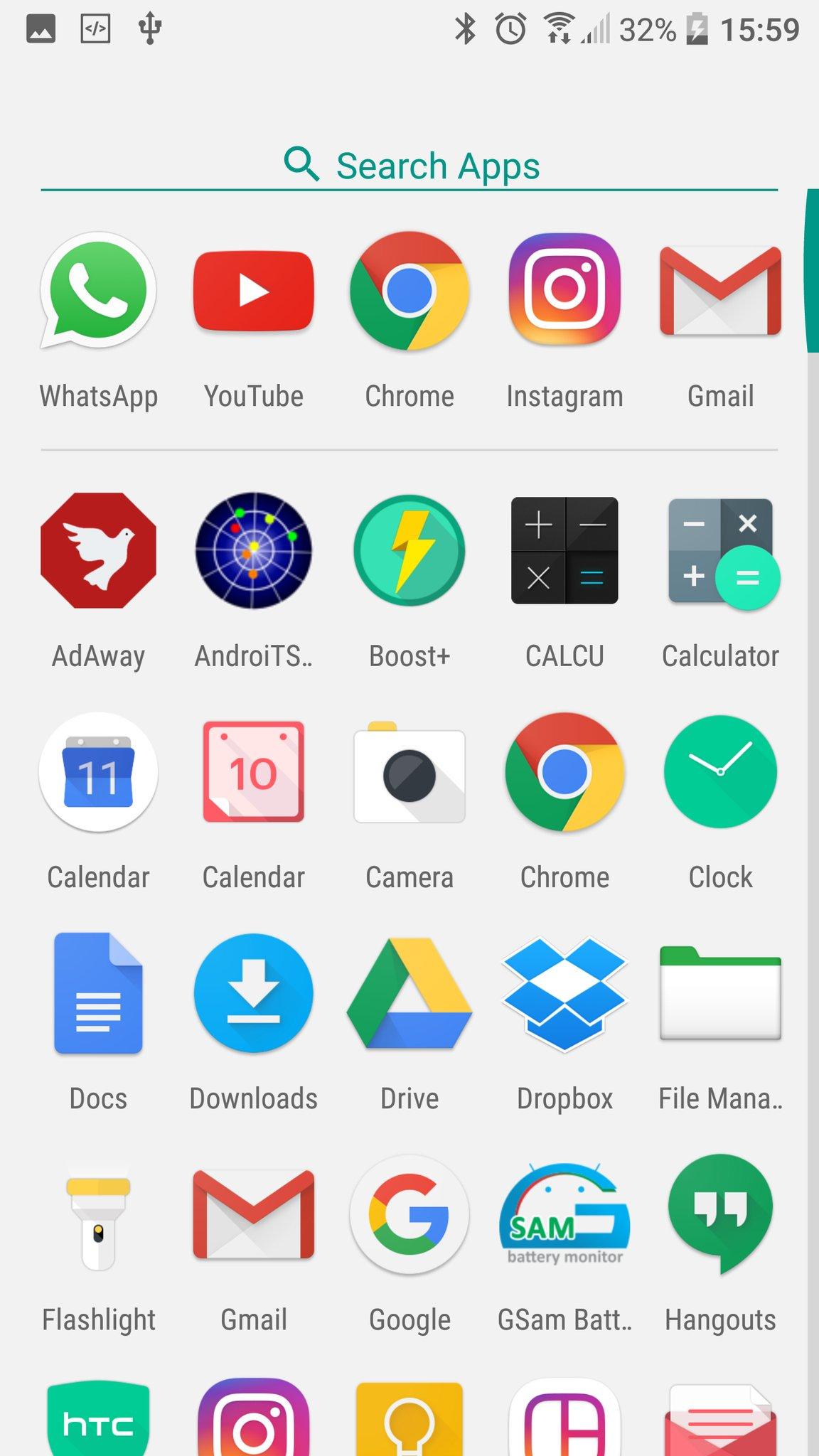Here is a detailed and cleaned-up caption for the screenshot of the phone:

---
Screenshot of a smartphone home screen showcasing various apps arranged in rows. At the top of the screen, the status bar displays several icons: a picture icon, a trident icon, Bluetooth symbol, alarm clock, Wi-Fi signal, battery percentage indicator, and the current time. Below the status bar is a light gray search bar that features a magnifying glass icon and the text "Search apps" written in turquoise, accompanied by a turquoise underline and scroll bar.

The home screen background is a very light gray. The first row contains five frequently used app icons: WhatsApp, YouTube, Chrome, Instagram, and Gmail. Directly beneath this row is a gray line separating the next set of apps: AdAway, Android, TS Boost (with a lightning bolt icon), Calculator, and another Calculator. Following this is another row listing: Calendar, Calendar, Camera, Chrome, and Clock.

Continuing downward, the next row includes: Docs, Download, Drive, Dropbox, and File Manager. Subsequently, the following row displays: Flashlight, Gmail, Google, GSM Battery, and Hangouts. At the bottom, there are a few more apps, partially revealed: HTC, Instagram (with only the icon visible), and a yellow light bulb icon. These might be additional frequently used or auto-suggested apps.
---